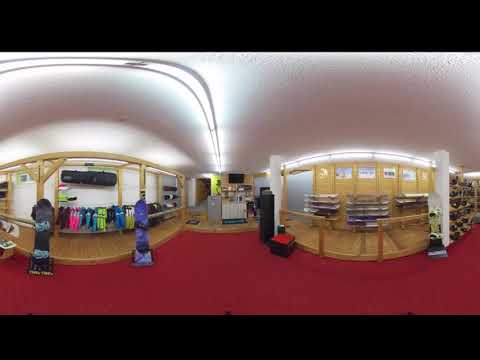This panoramic digital photograph captures the vibrant interior of a retail store, possibly specializing in snowboard equipment. The store features a white ceiling illuminated by bright lights, contrasting with the red carpeting underfoot. The walls are white with light wood-colored shelving and various wooden platforms or kiosks scattered throughout the space. Hanging racks and well-organized shelves display an array of products including snowboards, snow boots, and multicolored coats. On the left side of the store, two blue and green clothing displays stand out in front of a wall lined with coats, while further back, multiple shelves hold additional products. To the right, several racks showcase an assortment of snowboards, emphasizing the store’s specialty. People can be seen browsing the displays, enhancing the lively and dynamic atmosphere of the store.